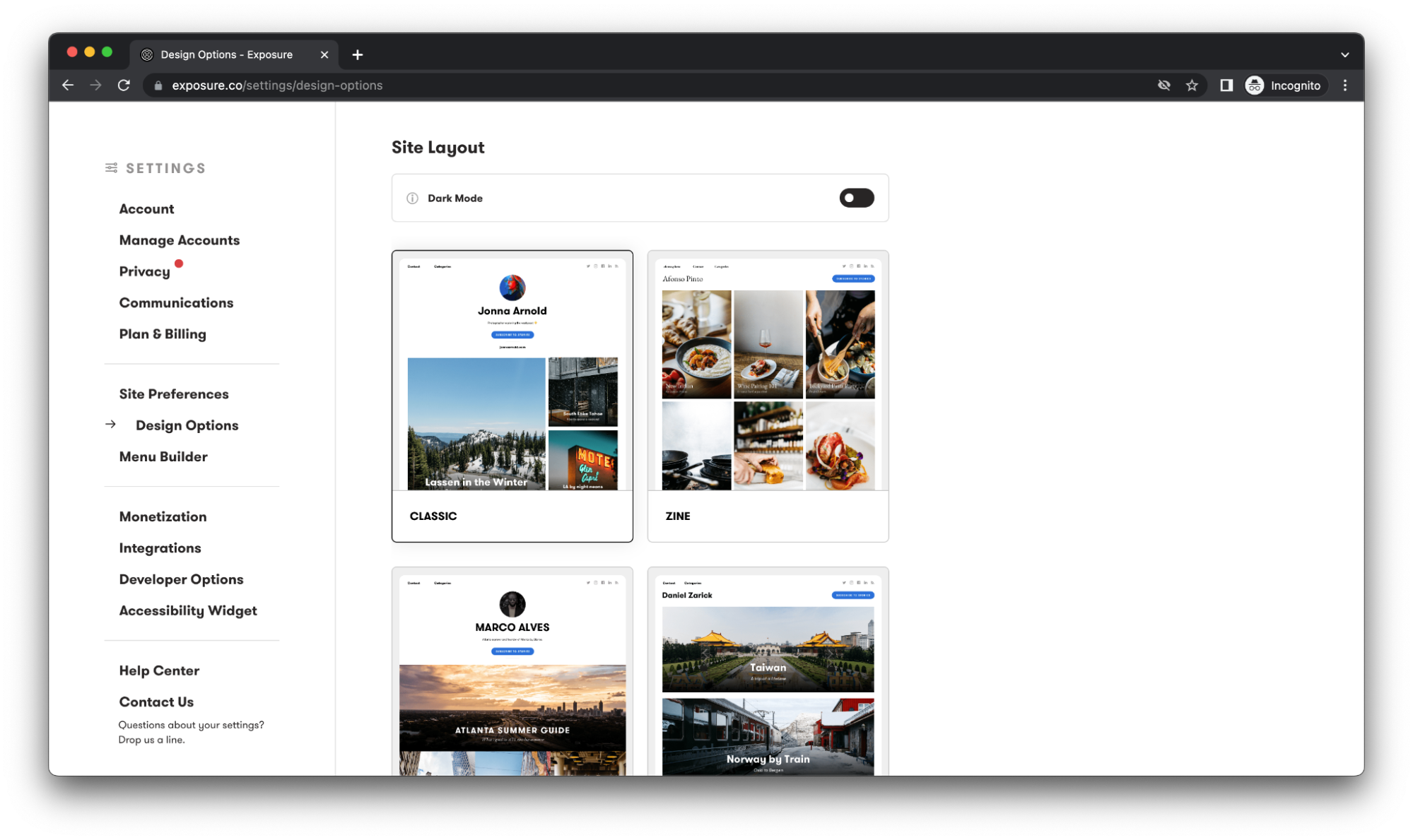Screenshot of a website showcasing various design and customization options. The upper left corner features the typical red, yellow, and green buttons for closing, minimizing, or maximizing the window. In the main content area, there are distinct sections labeled "Design Options" and another that appears to indicate "Exposure," although the small font makes it difficult to read clearly.

Below this section is a predominantly white interface with a vertical sidebar displaying an array of settings. These settings include:

- **Settings**
- **Account**
  - Manage Accounts
- **Privacy** (highlighted with a red dot)
- **Communications**
- **Planning and Billing**
- **Site Preferences**
- **Design Options** (tagged for emphasis)
- **Menu Builder**
- **Monetization**
- **Integrations**
- **Developer Options**
- **Assembly Widget**
- **Help Center**
- **Contact Us**

To the right, separated by a vertical gray line, there's a section titled "Site Layout," which contains clickable options for configuring the layout of the website. This section features various thumbnail images depicting different ways to stack and arrange pictures within the site layout, although the configuration options are currently turned off.